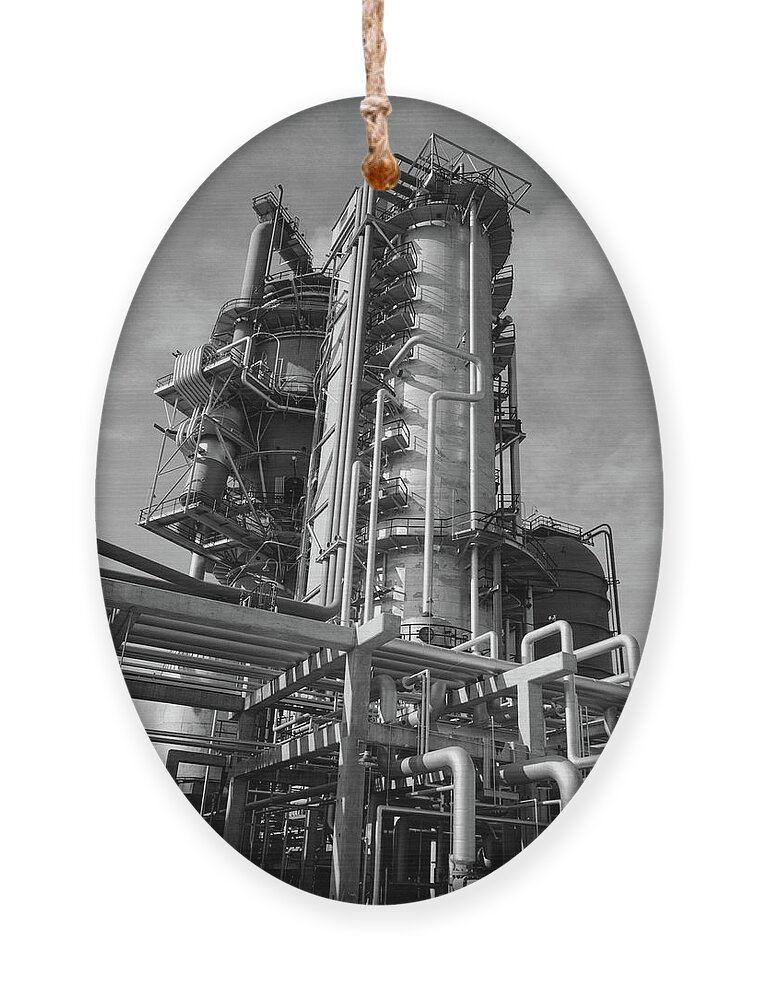This oval-shaped, photographic-style ornament features a black and white image of a 1960s crude oil distillation tower at an industrial plant. The tall, cylindrical metal tower is prominently placed at the center, boasting around ten sets of balconies running vertically along its side, offering a series of walkable bridges. Scaffolding wraps around the tower, emphasizing its height and complexity. To the left of the tower, a large pipe extends upward, adding to the intricate network of metalwork typical of industrial settings. The base of the image is dominated by numerous metal pipes supported by beams, creating a dense and visually engaging foreground. 

On the right side of the image, a roundish silo-type structure is partially visible, complementing the industrial theme. The background features a grayish tone, enhancing the stark contrast of the black and white photograph. The entire scene is captured within an oval frame, indicative of the ornament's design, which is intended to be hung, as evidenced by the rope or necklace element at the top of the image. This adds a unique touch, transforming an industrial photograph into a decorative piece without any accompanying text.